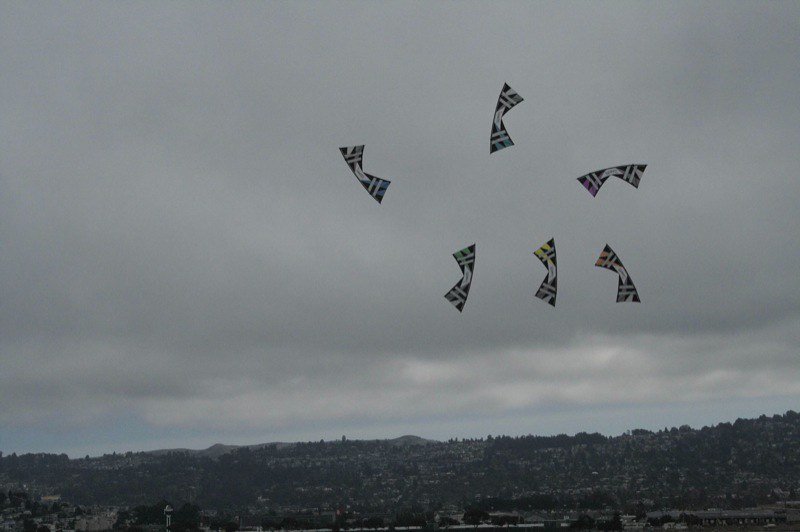In this grainy, slightly older photograph taken on a dull, cloudy day, six kites soar high in the sky against a backdrop of low hills dotted with indistinct structures that could be houses and trees, suggesting a rural area. The landscape orientation captures a gray sky with a faint strip of blue near the horizon. The kites, atypical in shape, each have two vertical stripes on their triangular points. The top right kite is purple, the top middle is a tealy green, and the top far left is a darker blue. The bottom kites include a slightly lighter tealy color, a yellow one, and an orange one on the bottom right. Despite their vibrant colors, the poor picture quality makes the details less discernible. No visible attachments are apparent on the kites, which are positioned closely together, floating over what appears to be shrubs and flat land that slopes slightly to the left.